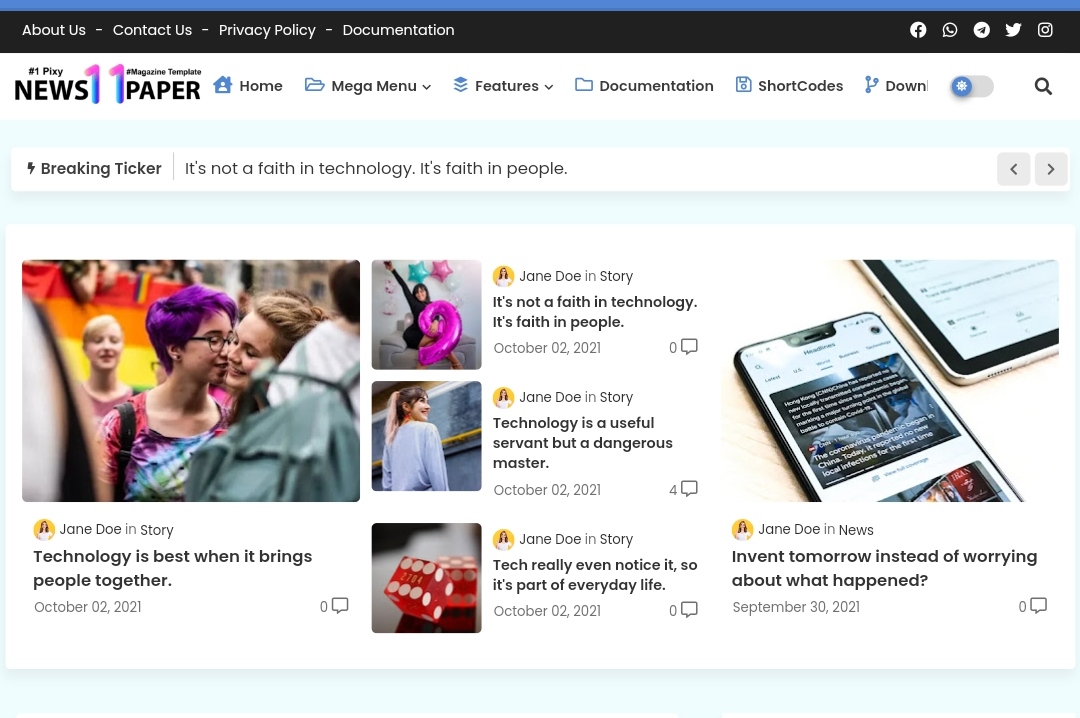At the top of the image, a blue horizontal rectangle serves as a header. Below this header, a much larger dark gray rectangle spans across the width of the image. On the left side of this dark gray rectangle, white text is displayed, while the right side features a series of white social media icons in the following order: Facebook, WhatsApp, Telegram, Twitter, and Instagram.

Beneath this gray section, the background turns white with the words "News 11 Paper" prominently featured. The number "11" is stylized in larger, colorful blue and pink digits, making it stand out more than the surrounding text. 

Below this, there is black navigation text arranged horizontally: "Home," "Mega Menu," "Features," "Documentation," "Shortcodes," and an additional menu item that appears to be cut off but starts with "Down." Each of these menu items is accompanied by a small blue icon to its left. 

Adjacent to the navigation menu is a blue slider icon depicting a sun, likely for toggling between light and dark modes. To its right is a black magnifying glass icon, presumably representing a search function. 

Further down, a white rectangle contains navigation arrows on the far right. Within this rectangle is an image of two girls, possibly at a Pride parade. The girl on the left has purple hair, while the girl on the right has brown hair. In the background, another girl looks toward them, and a vibrant rainbow flag is visible, enhancing the celebratory atmosphere of the event.